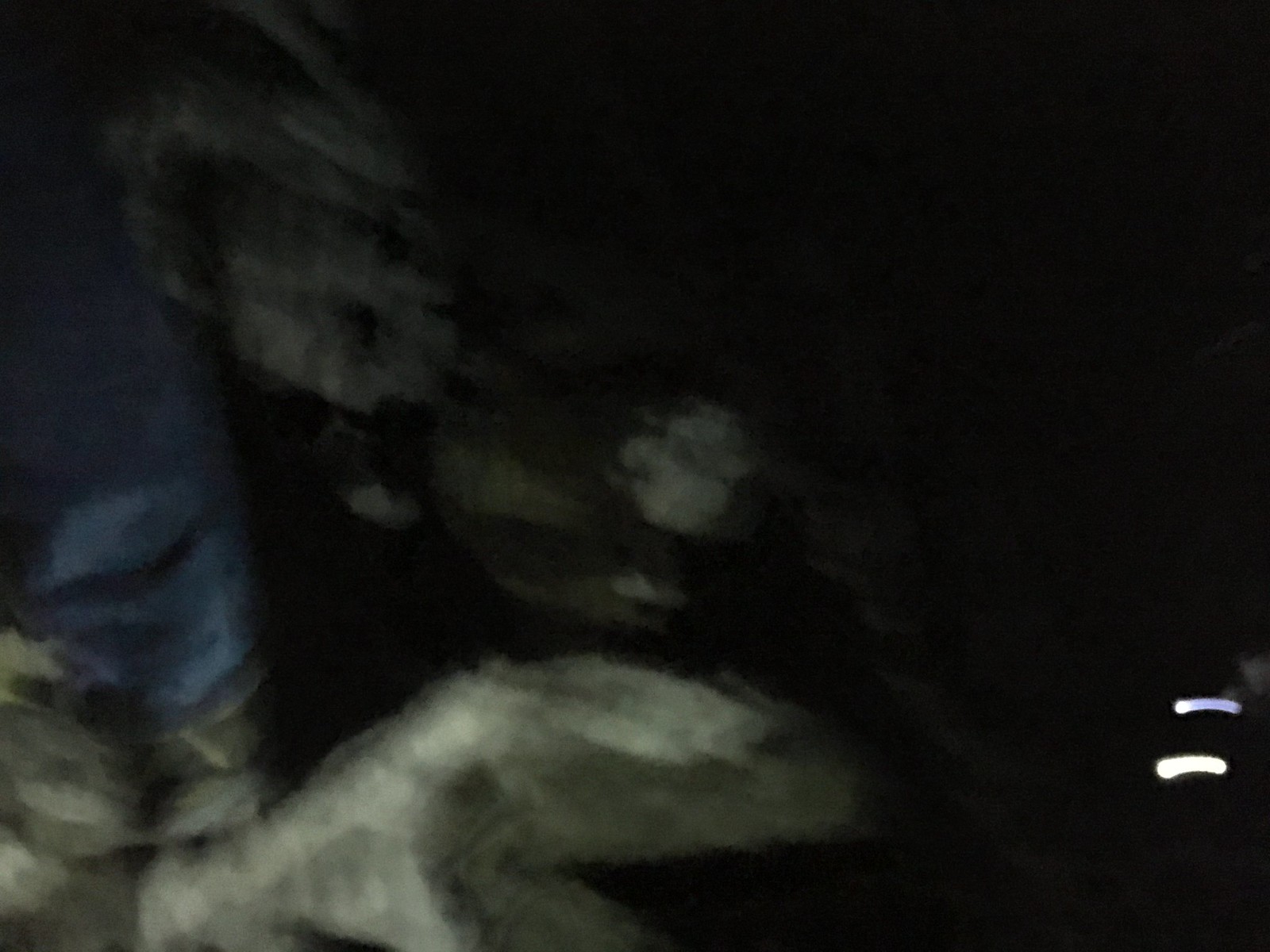A blurry nighttime photograph with a predominantly black background. In the bottom right corner, two horizontal neon lights pierce through the darkness. The lower part of the image features what appears to be a gray mitten, likely worn on a hand, showing a larger section at the top and a smaller V-shaped piece at the bottom. Attached to the mitten is a blue shirt, suggesting the presence of a person. The rest of the background consists of indistinct gray and white shapes, adding to the overall obscurity and mystery of the scene.